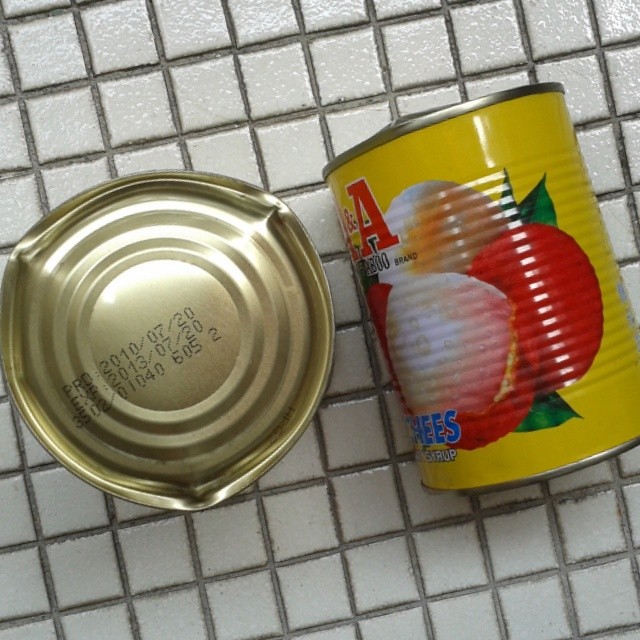In this image, you see two canned goods resting on a 1x1 inch white ceramic tile countertop with a standard gray grout. On the right, there's a can featuring a sunny yellow label adorned with images of fresh peaches complete with moisture condensation. The label has red lettering at the top and displays the letters "EES" at the bottom, likely indicating the brand or variety. The can is laid on its side, suggesting it could roll. To the left, there's a round lid which appears to have detached from the can. This bulging lid, with three indentations around the edge, features stamped text indicating a production date of "2010-07-20," an expiration date of "2013-07-20," and a batch code "3502-01040 6052."